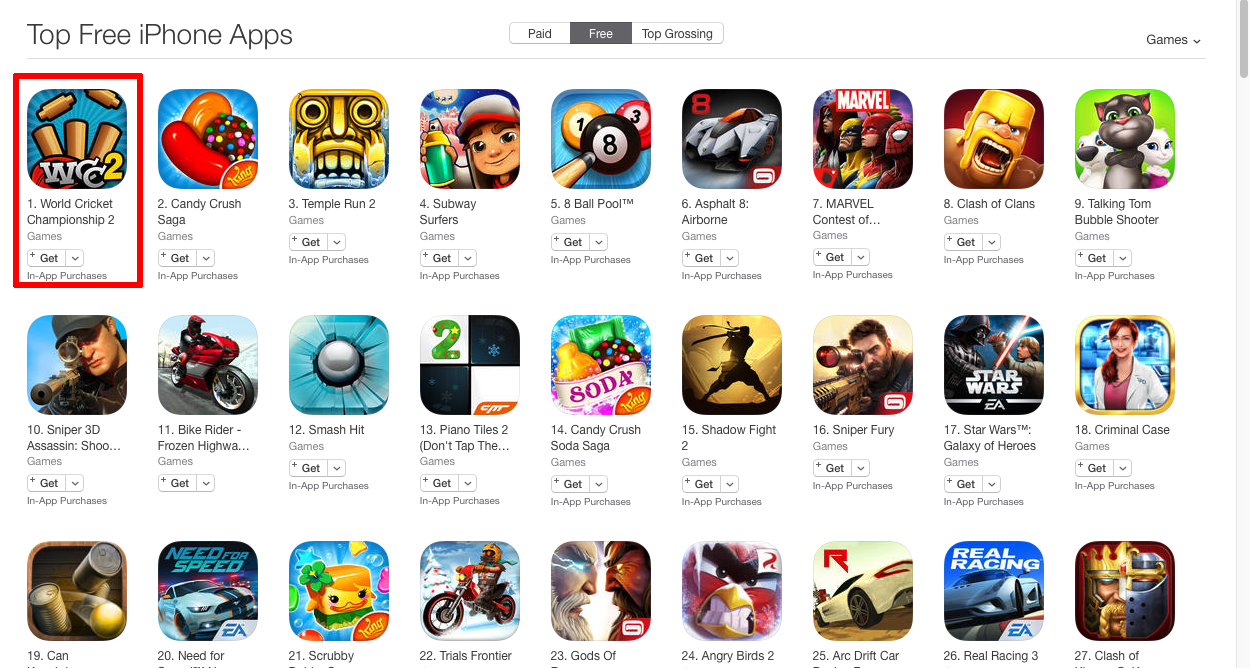The screenshot showcases a webpage enumerating the "Top Free iPhone Apps." The largest font, located in the upper left-hand corner, reads "Top Free iPhone Apps." Adjacent to this title are clickable buttons labeled "Paid," "Free," and "Top Grocery." The "Free" button is highlighted, indicating the current category. Displayed beneath are the top 27 free apps, organized into three horizontal rows with nine apps per row. Dominating the first spot is "World Cricket Championship 2," while the app ranked 27th, partially obscured, appears to be "Clash of Clans." The background of the page is predominantly white, providing a clean and minimalistic look.